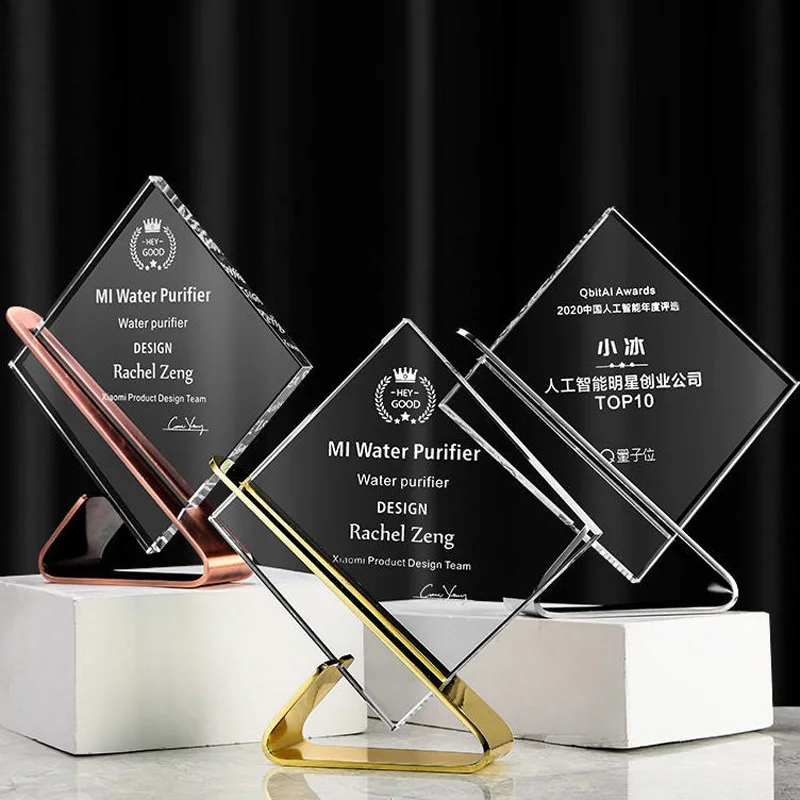The image captures three elegant glass awards with a rhombus-like, see-through shape, each mounted on differently colored metallic stands, positioned on a white concrete block. The central trophy, supported by a golden stand, reads "M.I. Water Purifier, Water Purifier Design, Rachel Zhang." To the left, a trophy with a pinkish stand bears the same inscription. On the right, a trophy on a silver stand features foreign text, along with the words "Top Ten." The backdrop is a dark black curtain, adding a formal touch to the awards setting.